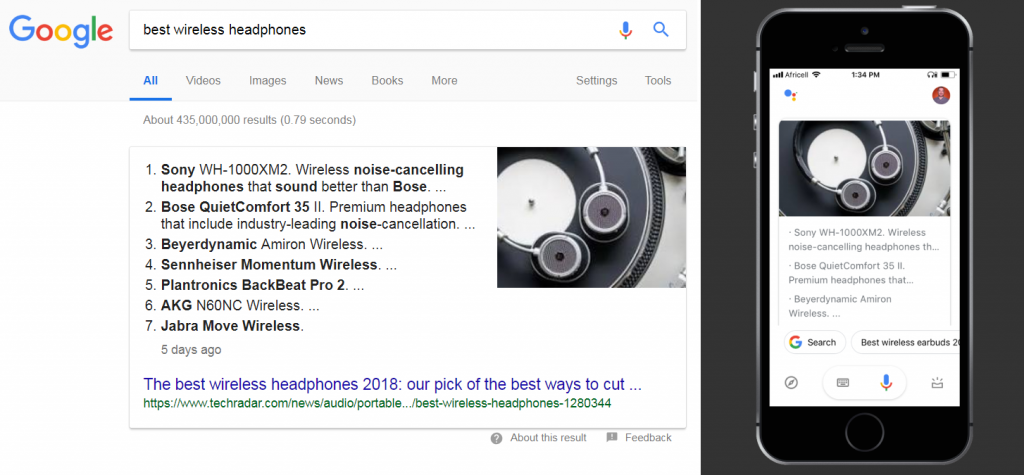The image is a split-screen comparison displaying search results for "best wireless headphones" on two devices: a laptop (left) and a smartphone (right). On the laptop screen, the Google search results indicate approximately 435 million results found in less than a second. The top-ranking headphones include:

1. **Sony WH-1000XM2** - Wireless noise-cancelling headphones praised for superior sound quality over Bose.
2. **Bose QuietComfort 35 II** - Premium headphones noted for industry-leading noise cancellation.
3. **Beyerdynamic** - Wireless headphones.
4. **Sennheiser Momentum Wireless**
5. **Plantronics BackBeat Pro 2**
6. **AKG N60NC Wireless**
7. **Jabra Move Wireless**

Beneath these listings, an article from TechRadar is highlighted, titled "The best wireless headphones 2018: our pick of the best ways to cut."

The smartphone screen on the right side of the image also shows search results, featuring detailed listings for the Sony WH-1000XM2 and Bose QuietComfort 35 II, consistent with the search results displayed on the laptop. The comparison effectively illustrates how the same Google search displays on different devices, providing a user-friendly view of top-rated wireless headphones.